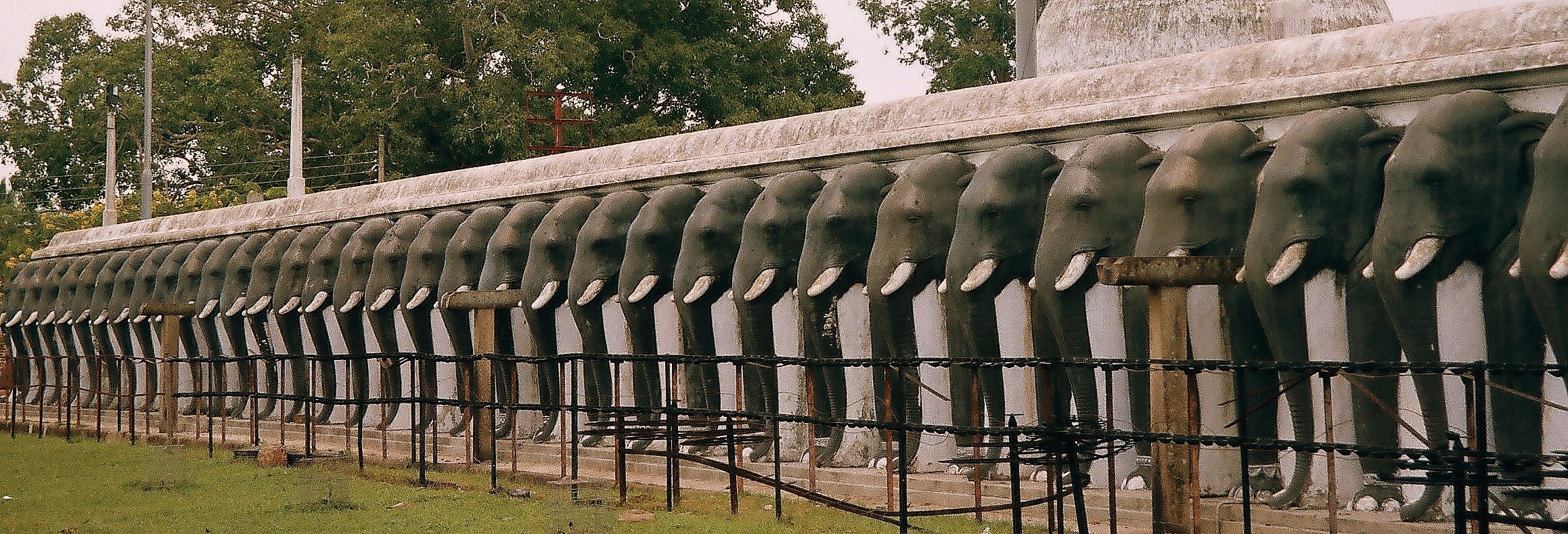The photograph captures a scene with green grass in the foreground, leading up to a black iron railing that borders the area. Behind the railing is a walkway covered in a tan or brown gravel, adding a distinct path in front of a row of life-sized elephant statues. The statues are intricately carved and painted to resemble real elephants, with grey bodies and white tusks. Each statue is identical, aligned in a straight line with only their front legs, trunks, and heads protruding from a large stone wall, giving the impression they are emerging from it. The wall appears to be part of an old or historic stone structure. Further details include occasional wooden posts set between the railing and the walkway, and in the background, trees rise up above the stone wall, adding a natural element to the scene.